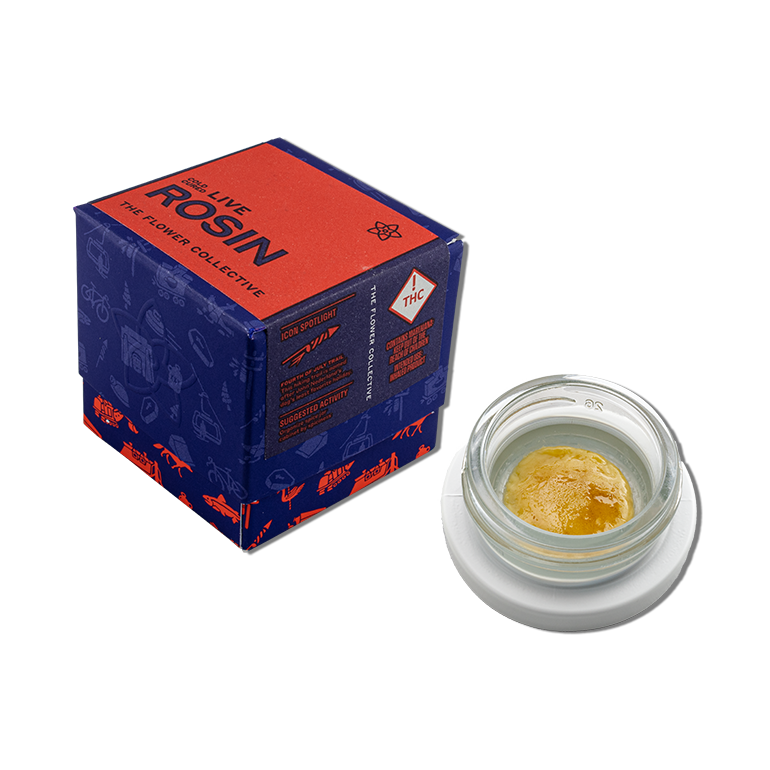The image showcases a carefully arranged product display featuring Live Rosin by The Flower Collective. Central to the scene is a blue box with an orange logo at the top, adorned with intricate depictions of fish, boats, and trains along its sides. The box is positioned at a slight angle, giving it a diamond shape from the viewer's perspective, and includes a clear THC warning label. Prominently displayed on the box is the name "Live Rosin, The Flower Collective," with a flower-like company logo above.

To the right of the box sits a small glass vial containing a yellow, wax-like substance with a texture reminiscent of applesauce, sitting atop a white base. The glass container, approximately the size of a quarter to a 50-cent piece, has its lid placed underneath it, and all elements in the arrangement are presented upright, ensuring each detail is visible and clear. The entire composition highlights the quality and detail of the Live Rosin product in a visually appealing manner.